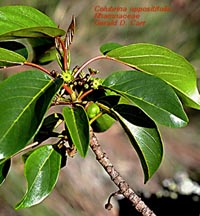The image depicts a small plant featuring a branch extending from the bottom right corner. The branch is characterized by a brown bark with blackish lines, resembling bark spots. This central stem, which has an orangish-reddish hue, holds together a collection of green leaves. The leaves are notably detailed; they are dark green with lighter lime green veins that create an intricate pattern. Some leaves appear to have tiny flower buds or the beginnings of fruit attached. The background of the image is blurred, suggesting an outdoor setting, possibly a forest, while sunlight appears to reflect off the leaves. In the right-hand corner, there is red text that seems to be the plant's identification in Latin, but it's too small and blurry to read clearly. The overall impression is one of a natural, vibrant plant against a subtly blurred backdrop.